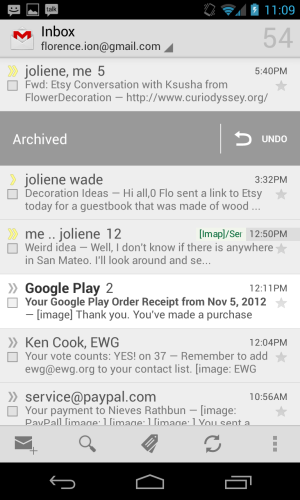This is a detailed description of an image captured from a smartphone inbox displaying various email threads. The prominent email address at the top is "florence.ion@gmail.com." Among the visible email threads, the first one mentions "Jolene, me," followed by the number "5." This email seems to be part of a forwarded conversation titled "Etsy conversation with Kusha from flower decoration," accompanied by a link "http://www.curiodicey.org."

As the viewer's eyes move down the image, an archived email is highlighted, featuring an "Undo" button with a circular arrow, indicating the option to reverse the archive action. 

Continuing the scan, another email from "Jolene" (or potentially "Jolene Wade") contains a subject or message snippet reading "decoration ideas hi-yah Flo sent a link to Etsy today for a guest book that was made of wood."

Further down, an email from "Jolene" is followed by another email from "Google Play to Ken Cook." Lastly, we can see part of an email from "service@paypal.com" with the subject line "Your payment to Neves Rathbun." The message preview reads, "You sent a," but it is truncated due to the image's dimensions.